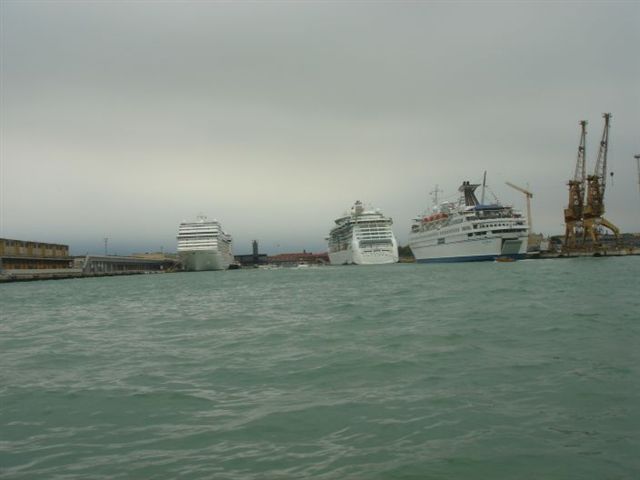This monochrome photograph captures a serene harbor scene, featuring a calm, greenish-gray body of water that occupies the bottom half of the image. The sky above is overcast and gray, lending a somber and misty atmosphere to the setting. To the left, there is a segment of a canal, framed by buildings that could possibly be hotels or other large structures. Dominating the center of the image are three substantial white ships, closely resembling cruise liners with visible portholes hinting at passenger rooms; one ship appears to be docking, its front angled as if preparing to open. On the right side of the photo, several tall yellow cranes, equipped with hooks, stand prominently against the skyline, ready for loading and unloading activities. The muted color palette of the scene, from the grayish sky and water to the white ships, emphasizes the quiet and industrial nature of the harbor.